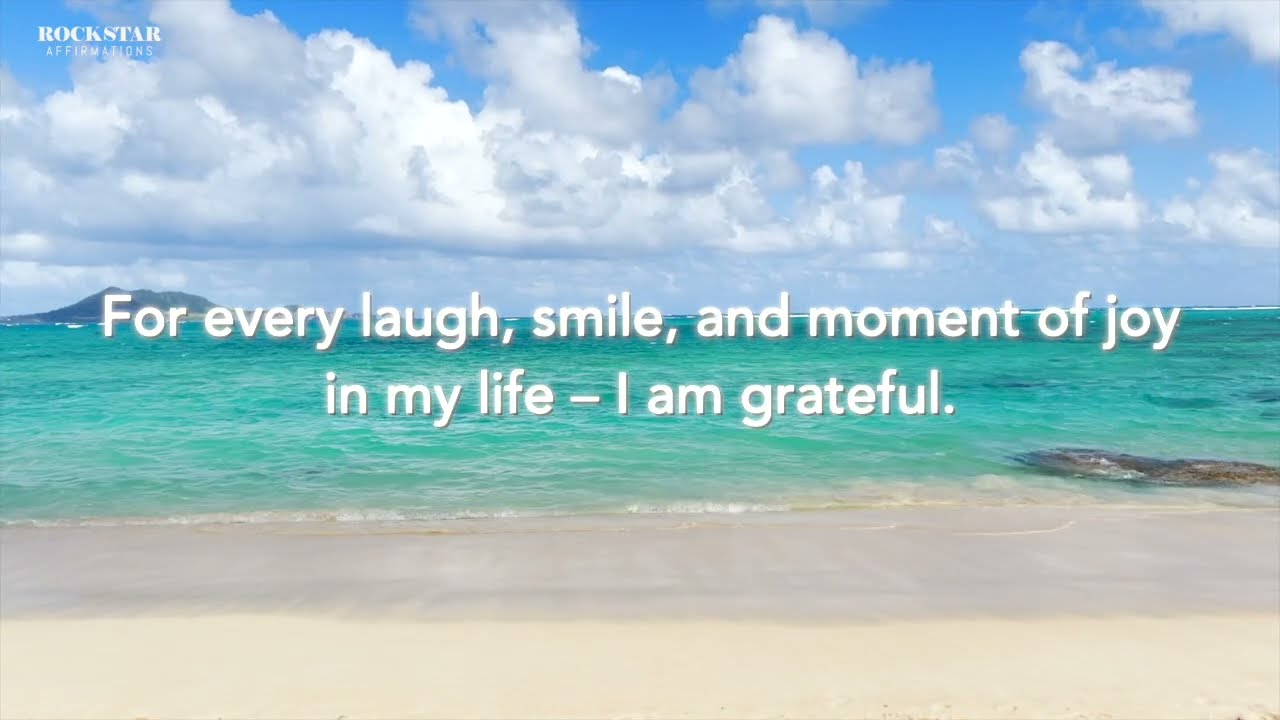The image is a serene photograph of a tropical beach scene divided into three horizontal sections. In the foreground, there is a combination of dry and wet sand, gently caressed by calm waves. The middle ground features blue, turquoise waters stretching out to a distant, barely noticeable horizon line. On the left side, far in the distance, there's a hint of an island or mountain jutting up, while smaller rocks and coral peek above the water to the right.

Above this tranquil scene, the sky is a stunning blue adorned with clouds, adding to the picturesque quality of the landscape. Text overlays the image: in the upper left corner, the logo "Rockstar Affirmations" is visible, and centrally placed is a larger, white, glistening font that reads, "For every laugh, smile, and moment of joy in my life, I am grateful." The composition and the message together exude a sense of peace and gratitude.